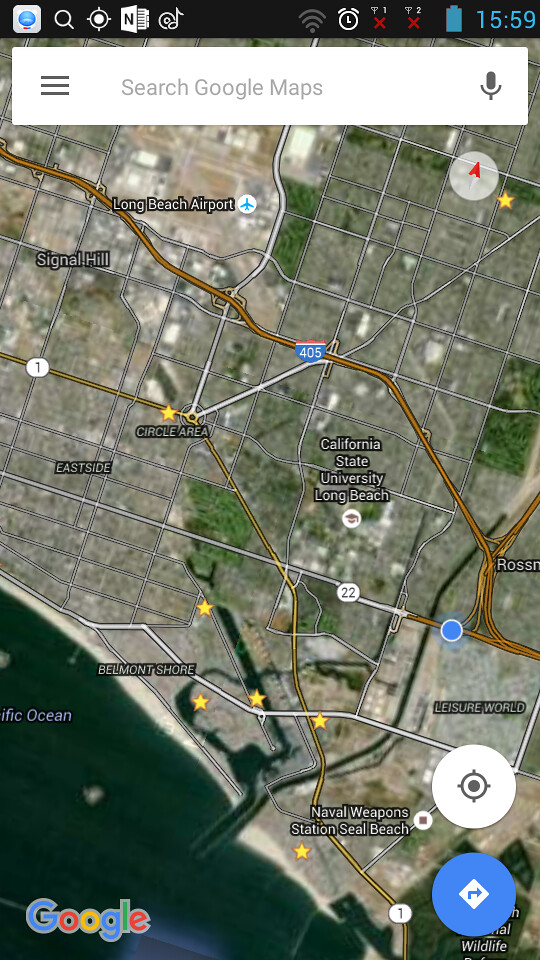This satellite image, captured from Google Maps, showcases a detailed view of the Long Beach area in California. At the topmost edge of the screenshot, there are standard cell phone screen icons displaying battery power, time, and other typical indicators. Immediately below these icons is the white Google Maps search bar, featuring options for a typed search or an audio search, denoted by the microphone symbol.

Central to the image is the satellite overlay highlighting several prominent landmarks, including Long Beach Airport, Signal Hill, California State University Long Beach, Naval Weapons Station Seal Beach, and Leisure World, among others. Some of the names appear slightly blurred and unclear, but they collectively point to a location within California.

In the lower left corner of the image, the distinctive Google logo—shown in its customary colors of blue, red, yellow, blue, green, and red—can be seen superimposed over the ocean. The bottom right corner features a blue circle containing a white diamond with a right-facing arrow, alongside a white circle with a bullseye at its center.